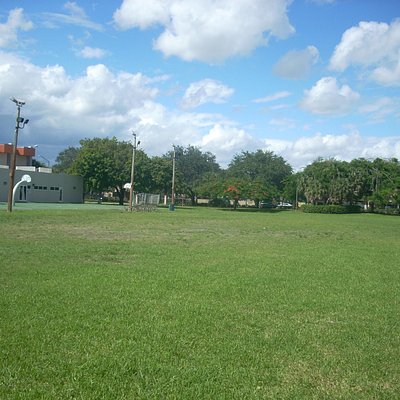The image captures a large, open green field of grass, part of which appears slightly dried with patches revealing some brown or dirt. The lush field extends to the forefront, suggesting a spring or summer setting. Dominating the upper part of the image is a vast, blue sky filled with fluffy white clouds, with hints of a possible rain cloud to the left. In the left background stands an ambiguous grayish building with orange, reddish tops, potentially serving various purposes such as storage, retail, or academic facilities. This building is flanked by three tall electrical poles and a few lights, possibly cameras, overseeing the area. A white basketball hoop is visible beside the building. Dense rows of trees and some bushes populate the middle and back portions of the scene, reinforcing the verdant, serene atmosphere. It's a bright day, and the elements together evoke the tranquil ambiance of a park or open recreational space.